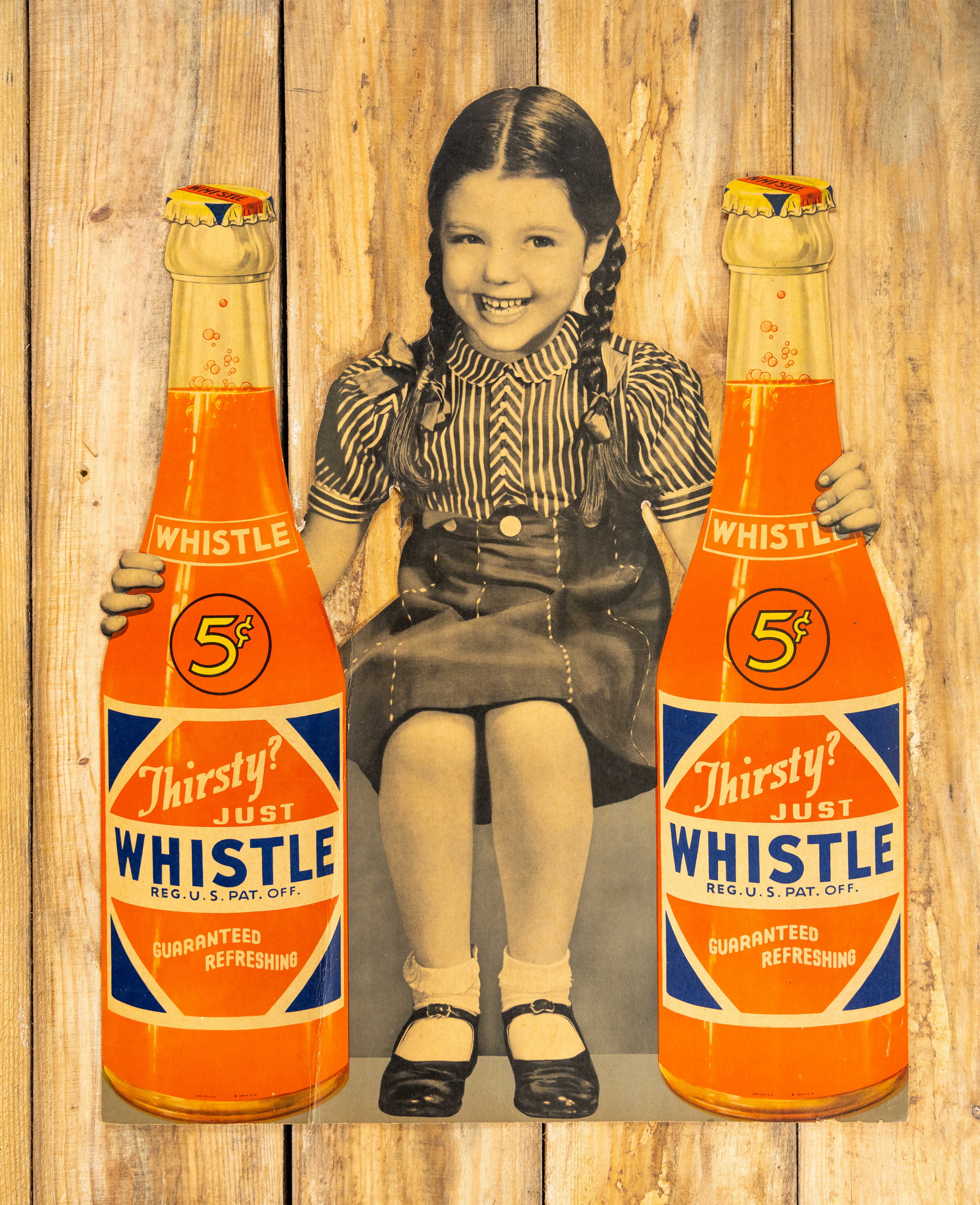The photograph showcases a vintage promotional signboard for a drink, prominently featuring a young girl in a black-and-white cutout. She is cheerfully holding two identical glass bottles filled with an orange liquid, each bottle placed on either side of her. The bottles are adorned with several lines of text reading: "Whistle," "Five cents," "Thirsty? Just Whistle," "Reg. U.S. Pat. Off.," and "Guaranteed refreshing." Each bottle has a yellow and orange bottle cap. The girl, wearing a short skirt, white socks, and shiny black Mary Jane shoes, is depicted with braided pigtails and a black-and-white striped shirt, smiling widely. The rectangular signboard is placed on a flat wooden surface with visible gaps between the wood panels, enhancing the rustic feel of the advertisement.